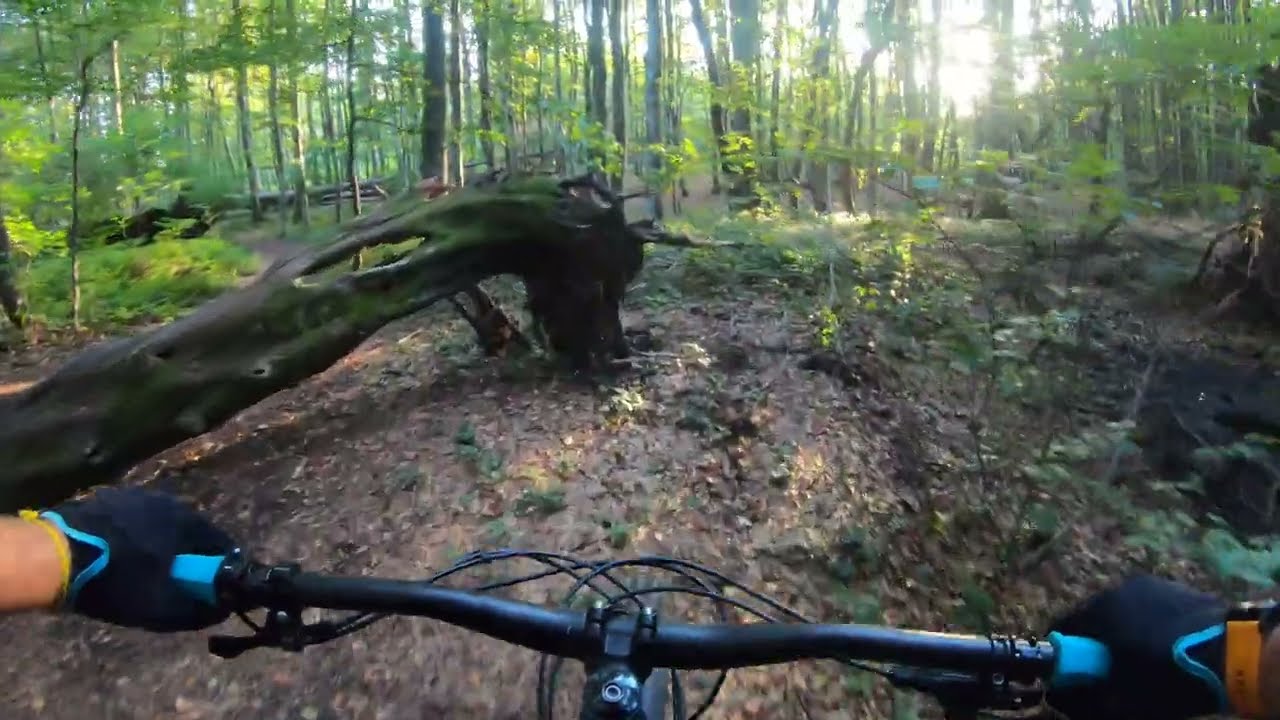Taken from the perspective of someone riding a mountain bike on a bright, sunny day in the woods, this photograph offers a vivid view ahead. The rider’s black-gloved hands, gripping sturdy black handlebars accented with light blue grips, are positioned in the bottom right and left corners of the image. A watch with an orange wristband adorns the right wrist, and a thin yellow bracelet circles the left. The rough, uneven ground looks muddy and bumpy, with sparse vegetation. On the left side of the frame, a fallen tree trunk covered in green moss, several feet in diameter, lies prominently. In the background, a forest of tall, thin trees with bright green leaves stretches upward, creating a canopy that allows sunlight to stream through, particularly noticeable in the upper right portion, indicating it's either late in the day or the sun is low. The photograph captures the stillness of the forest interrupted only by the motion blur at the edges of the frame, suggesting the rider’s movement through this rugged, tranquil woodland trail.